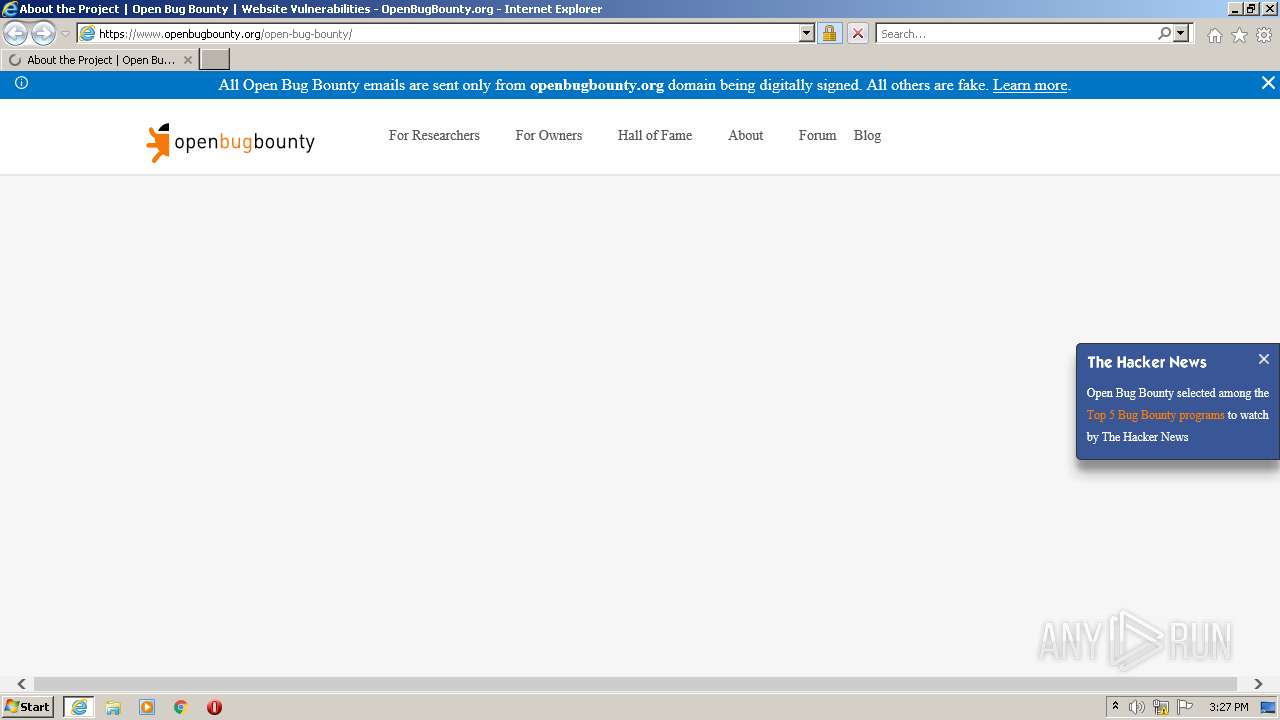This is a detailed screenshot of a desktop website viewed in Internet Explorer. The familiar blue Internet Explorer bar at the top features the classic 'e' logo, with text in white for "About the project," "Open Bug Bounty," "Website Vulnerabilities," "Open Bug Bounty," and "Internet Explorer." On the right side of this bar are the gray control buttons for minimizing, maximizing, and closing the window.

Below the bar, there's a gray banner horizontally spanning the top, containing a white search bar alongside the Internet Explorer logo. The URL displayed is "https://www.openbugbounty.org/open bug bounty" in the address bar. Below this, there is an additional section with a drop-down menu for the web address, a lock symbol, a red X icon for stopping a web request, and another search box.

The active webpage tab reads "About the Project" followed by "Open Bug..." with no other tabs currently open. Directly beneath the tabs, a small blue banner indicates, "All Open Bug Bounty emails are sent only from openbugbounty.org domain being digitally signed. All others are fake," with an underlined "Learn more" link.

Further down, a wider banner with the "Open Bug Bounty" logo in black and orange is visible, accompanied by navigation links for "Researchers," "For Owners," "Hall of Fame," "About," "Forum," and "Blog." The rest of the webpage is shown as an empty gray area.

At the bottom of the screen, the Windows Start menu is positioned on the lower-left corner, adjacent to desktop icons for Internet Explorer, Media Player, Google Chrome, and an 'I' symbol for information. On the far right of the taskbar, recognizable icons such as the time, volume control, a white flag indicating system messages, and two upward-facing arrows representing additional hidden icons are present.